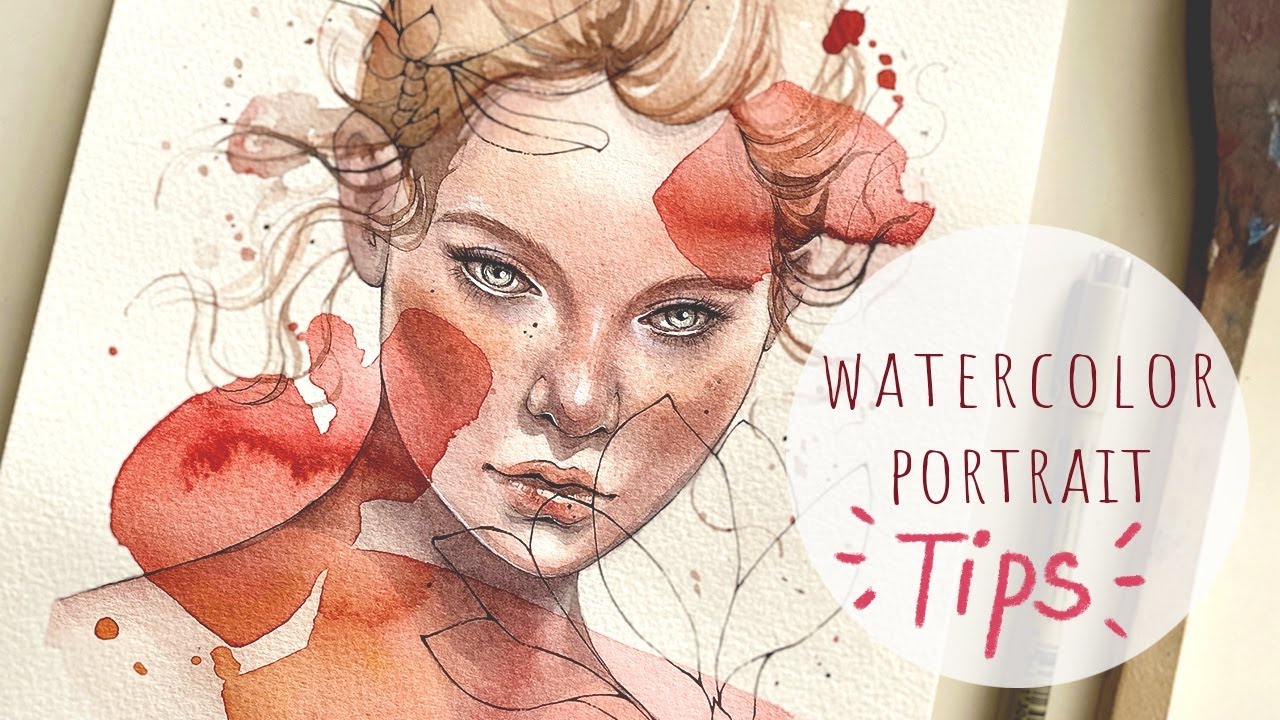The image is a landscape-oriented watercolor portrait of a young woman, showcasing her from the neck up. The subject is a white woman with light brown hair styled in a bun, with some locks waving at the sides as if blown by the wind. Her light eyes and delicate features are depicted primarily using fine ink pen or marker for the outlines, while the face and hair are vividly colored with watercolor, resulting in random reddish splotches that add an artistic and expressive touch to the portrait.

In the bottom right corner of the image, there is a prominent white circle containing text. The words "WATERCOLOR PORTRAIT" are displayed in all capital letters in a dark burgundy or maroon hue. Below this, the word "tips" is written in red, resembling colored pencil, with dashed lines emphasizing it, reminiscent of hand-drawn marks. This circle suggests that the image might be advertising watercolor portrait techniques or tips, possibly as part of a social media post or video tutorial. The overall presentation is both artistic and instructional, combining sketch and painted elements to highlight the beauty and technique of watercolor portraiture.